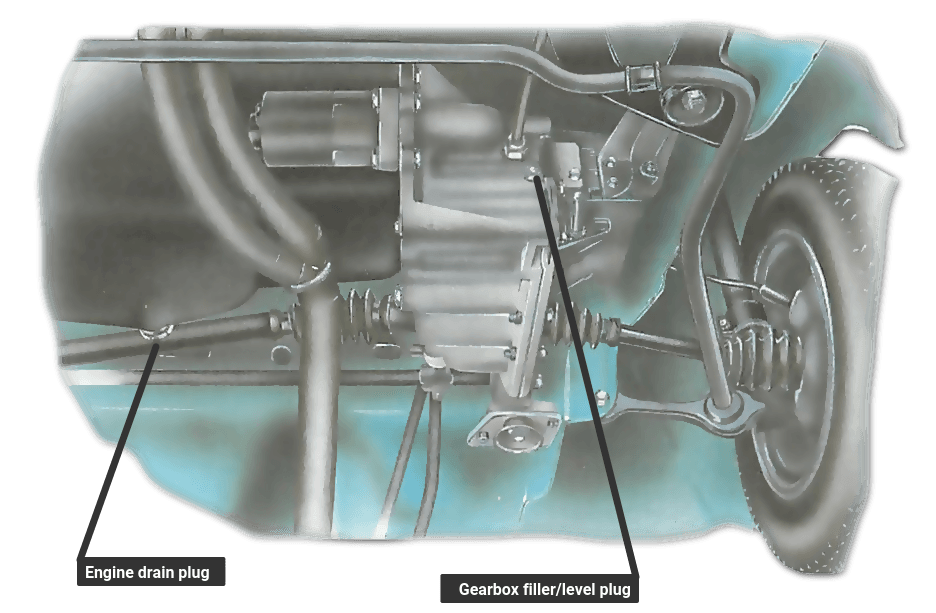This detailed illustration depicts the underside of a turquoise-teal car, highlighting various mechanical components in shades of gray and black. On the right-hand side, a partially visible wheel and axle can be seen, along with intricate metal connectors, screws, plugs, and pipes splayed throughout the undercarriage. A black pipe stretches horizontally on the left. The image includes two annotations: one black line traces from a black rectangle marked “Engine Drain Plug” in white text, pointing towards a specific plug on a pipe. Another annotation features a black arrow pointing downwards to the right from a black rectangle labeled “Gearbox Filler/Level Plug” in white text, directing towards a metallic box-like structure. The setting appears to be outdoors, given the graphic style and detailed emphasis on the car's mechanical layout.